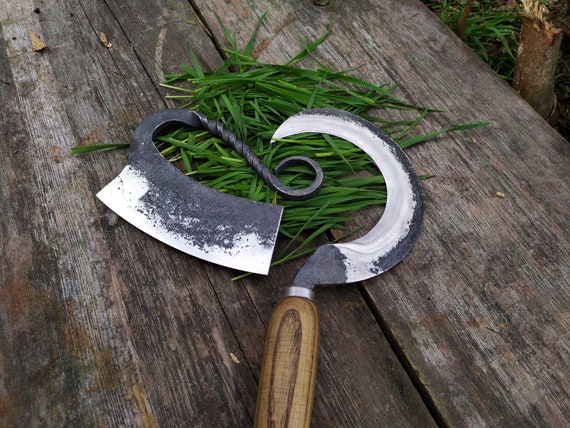In this outdoor color photo, the focus is on two well-used gardening tools laid side by side on a worn, grayish wooden table, which has various stains. Among cut greenery, likely grass or shoots, the tools stand out with their distinctive designs and heavily worn blades. The first tool is a wooden-handled scythe, approximately 12 inches long, featuring a sharp, silver blade with black accents. To its left, there is a second tool with a uniquely curved wrought iron handle resembling an 'S' shape, also bearing a sharp, silver blade. Both tools display significant wear, evident in the white, almost bleached appearance of their cutting edges, contrasting with their original grayish metal. The background shows a touch of greenery in the top right corner, indicating the setting might be near a field or grassy area.